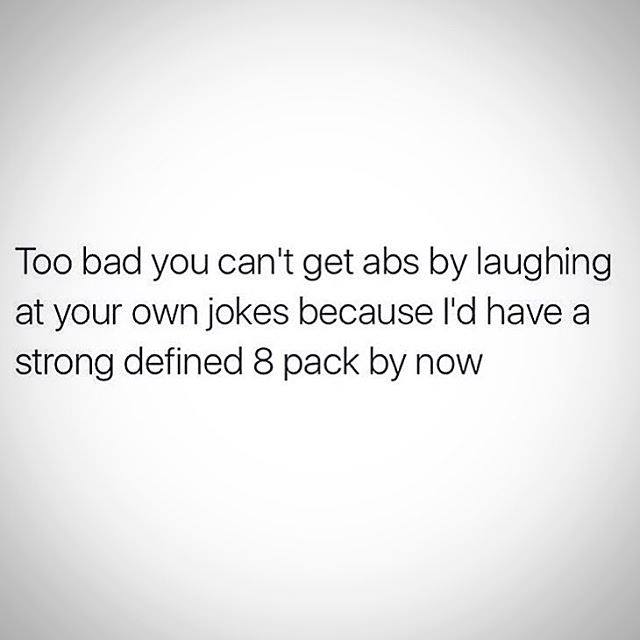The image is a square with a background that transitions from a darker gray at the corners to a lighter gray in the center. Positioned in the middle is a centered, three-line text in bold black font on the lighter gray section. The text humorously states, "Too bad you can't get abs by laughing at your own jokes because I'd have a strong defined 8-pack by now." The image is clean and simple with no additional figures or decorations, emphasizing the satirical nature of the message, likely intended as a shareable meme for social media.